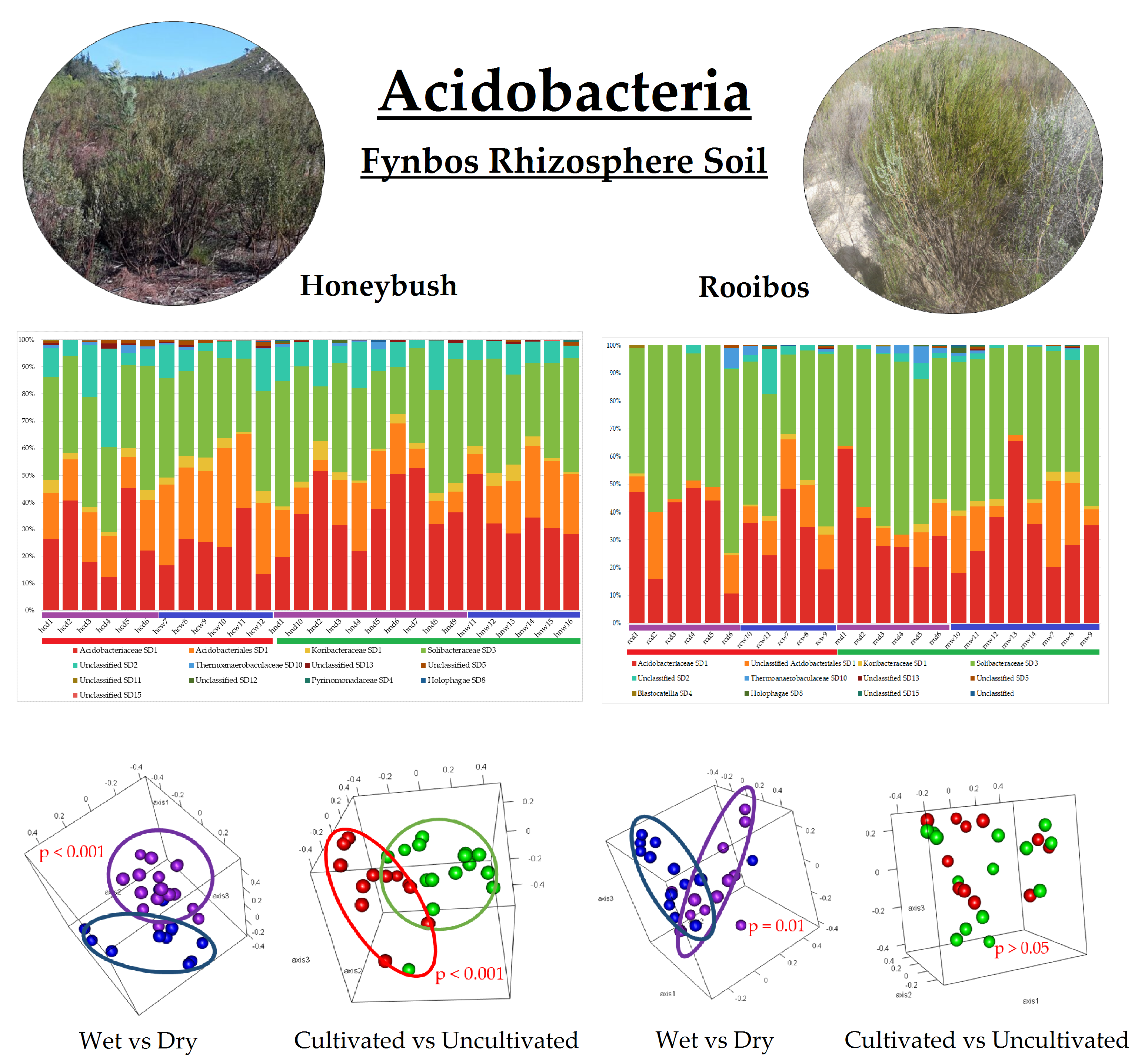The image prominently features a detailed presentation of various graphs and photographs, cohesively titled "Acidobacteria" in large black font with the subtitle "Fynbos Rhizosphere Soil" beneath it. Framing either side of the title are two circular photographs: the left labeled "Honeybush" and the right labeled "Rooibos," both displaying herbs growing in what appears to be arid, outdoor environments. Directly below these photographs are two distinct bar graphs, each with colored columns in teal, green, orange, and red, detailing data too small to read clearly but suggestive of various measured parameters.

Underneath the bar graphs are four three-dimensional scatter plots shaped like cubes. These graphs have X, Y, and Z-axes and are labeled as follows: the first is "Wet versus Dry," the second "Cultivated versus Uncultivated," the third again "Wet versus Dry," and the fourth "Cultivated versus Uncultivated." The scatter plots consist of dots in multiple colors, including purple, blue, red, and green, indicating different data sets or parameters related to soil conditions or bacterial presence. The arrangement of graphs and photographs provides a comprehensive visual analysis of Acidobacteria in the Fynbos Rhizosphere Soil under varying environmental conditions.